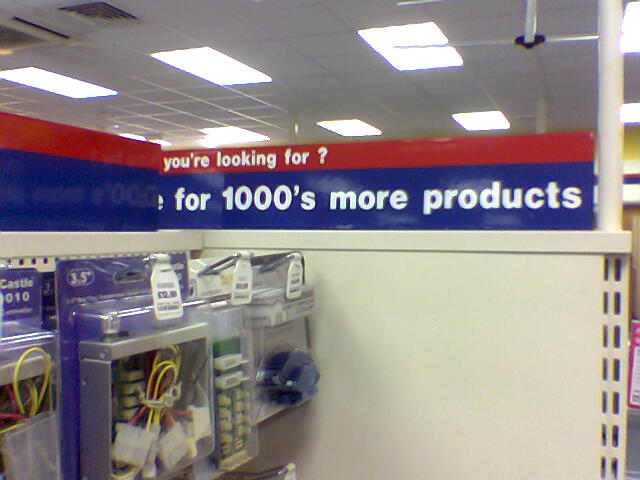This color photograph captures the interior of a hardware store, revealing a white-tiled ceiling adorned with rectangular fluorescent lights and visible air ducts. The focus is on a corner shelf festooned with a prominent red and blue banner stating, "Looking for more? Discover 1,000s more products." The shelf itself, painted white, displays an assortment of items, primarily wiring components and connectors in clear plastic cases. These products, which are possibly computer components, include red, yellow, blue, and green cords secured within transparent plastic bins. Additional wiring in various packages, including a blue box marked down to $2, can also be seen. To the left of the shelf are stacks of plastic containers, possibly holding metal squares, further emphasizing the store's extensive inventory.